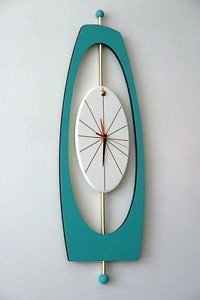This image features a retro, space-age wall clock reminiscent of the 1950s or 1960s design aesthetic, similar to styles seen in "The Jetsons" cartoon. The clock's face is situated within a central oval, which is held by a silver support. This support is capped with aqua-colored spheres at both the top and bottom. Surrounding the central oval is an outer frame that combines an oval shape with a squared-off bottom, all finished in a vibrant aqua color. The design exudes a groovy, mid-century modern vibe with its futuristic and playful elements.